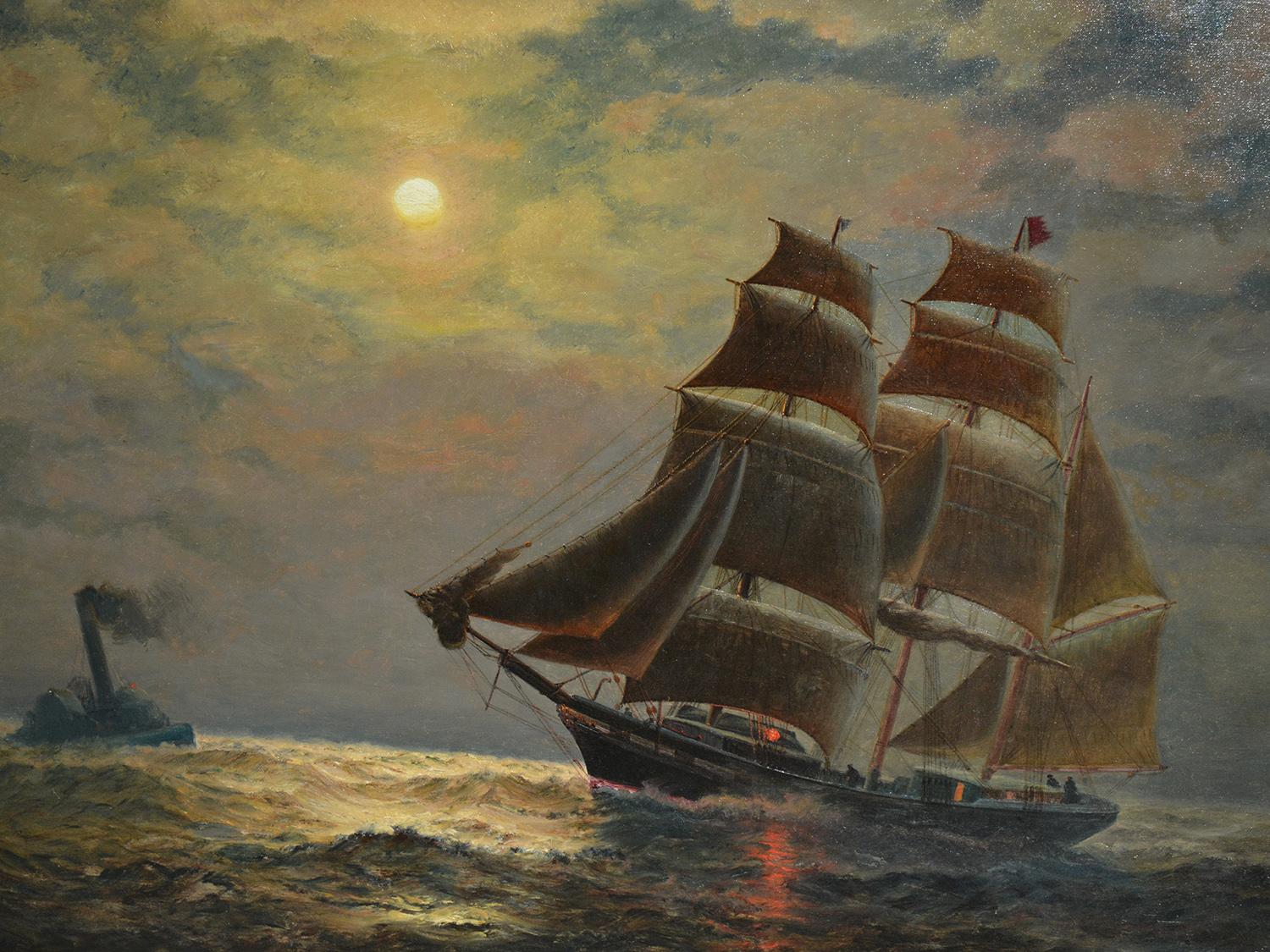The painting captures a dramatic maritime scene during what seems to be an evening with an impressionistic style. Dominating the composition is a large sailing ship with three imposing masts and numerous sails, the fabric appearing brownish under the moonlit sky. The ship, moving from the right side toward the left, has a lit cabin, casting a warm glow amidst the surrounding darkness, and revealing silhouettes of workers on the deck. To the left, a steamboat is depicted partially submerged, with smoke billowing from a smokestack, suggesting it's in distress. The choppy waters reflect the yellowish light of a high moon, casting a surreal glow on the scene. High waves and a visible red light on the ship amplify the sense of turmoil. A flag is noticeable on one of the central masts, adding a touch of realism to this evening seascape, rich in detail and movement.